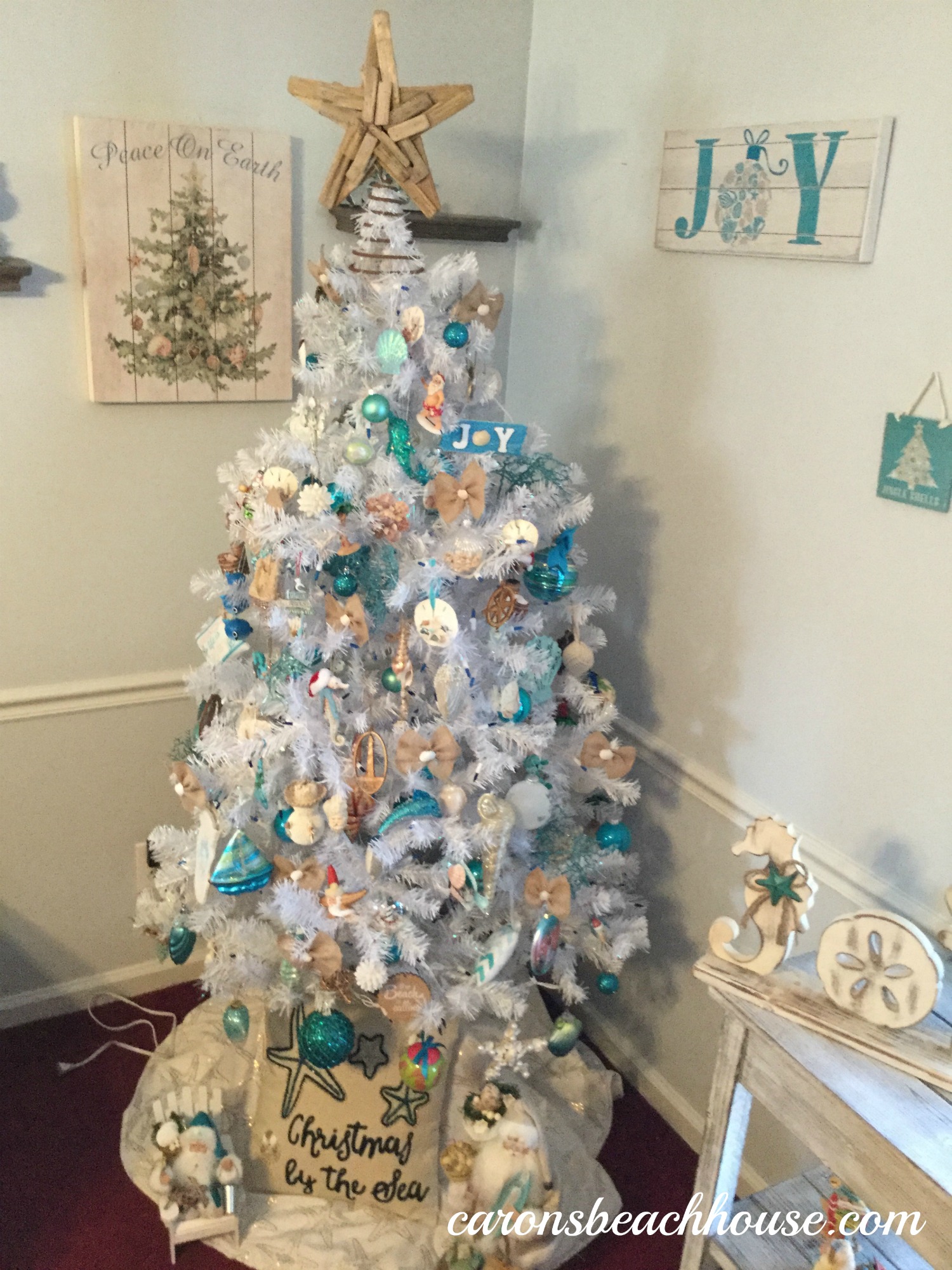In the corner of a room with white walls, stands a strikingly artificial white Christmas tree. The tree, made entirely of white plastic needles, is adorned with a nautical theme, featuring ornaments in shades of blue, tan, white, and darker teal. These include seashells, sand dollars, a sailboat, and various toys, alongside conventional Christmas bulbs. At the top of the tree, a large wooden star, appearing to be crafted from driftwood, is attached to the tree by a metal coil.

Beneath the tree, a pillow embroidered with three starfish bears the inscription "Christmas by the sea," and a white cloth is wrapped around the base. Adding to the festive setting, a Santa doll dressed in blue sits in a chair beside the pillow. The red floor provides a vibrant contrast, and in the bottom right corner of the photo, a URL, "kiernsbeachhouse.com," is inscribed in cursive. The walls also feature holiday-themed decorations, including framed pictures—one depicting a Christmas tree with the phrase “Peace on Earth” and another that says “Joy,” where the 'O' is shaped like a Christmas ornament.